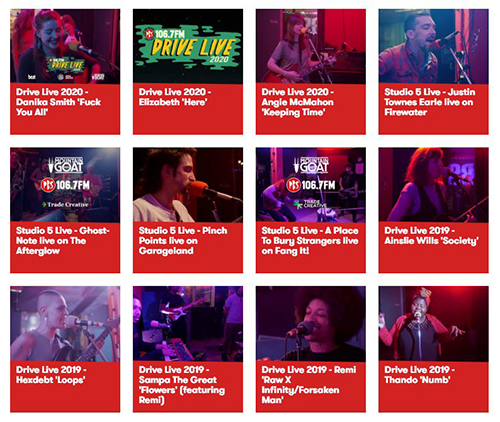This image consists of twelve individual squares, each containing a unique upper half and a red lower half. The lower part of each square features a distinct white inscription. 

One square showcases a man passionately singing into a red microphone, wearing a red checkered shirt. The lower red section states, "Studio 5 Live, Justin Townes Earl Live on Firewater."

Another square features a man with a big afro, singing with his eyes closed and a smile on his face. The caption on the red portion says, "Drive Live 2019 X Infinity Forsaken Man."

In a different square, there is a woman smiling and speaking into a microphone. She sports large green earrings and her hair is tied back with a pink scrunchie. The text below reads, "Drive Live 2020 Danica Smith, fuck you all."

One of the squares displays abstract green and black background imagery, with yellow text that reads "Drive Live 2020."

Each square collectively depicts moments of musical performance and personal expression, framed by the consistent red lower halves adorned with descriptive white text.